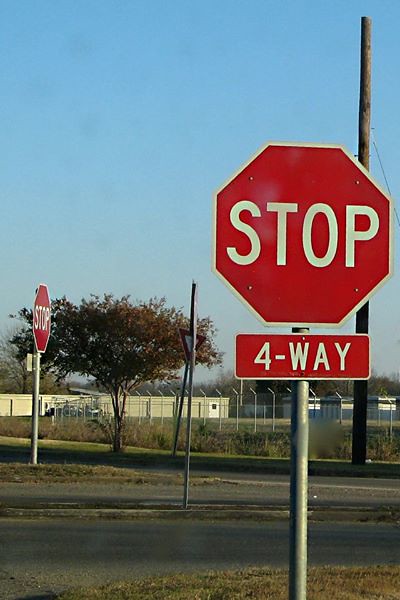The image captures a detailed scene of a four-way intersection under a clear blue sky. In the foreground, on the right side, stands a prominent red octagonal stop sign mounted on a round silver metal pole. This sign features the word "STOP" in large white letters with an additional small rectangular sign below it that reads "FOUR-WAY" in white letters. Adjacent to this stop sign lies a brown grassy area followed by a one-lane road. Noteworthy is the center concrete median of the intersection, which bears a vertical pole missing its signage.

To the left, another stop sign is visible at an angle, characterized by its slender steel pole and standard red and white "STOP" marking with no additional signs. This area is further defined by a combination of a barbed wire fence, a metal chain-link fence, and a large power pole. 

In the mid and far background, a single-story silver building extends from the left towards the center, accompanied by a trio of small gray storage buildings encircled by a chain-link fence. Not far from this building is a noteworthy YIELD sign mounted on a steel pole, featuring a red outer triangle and a white inner triangle, alongside a lush green tree and additional vegetation. 

Overall, the scene is rich with details of both the man-made elements, such as roads and signage, and the natural elements like trees and grass, all under a picturesque sky that completes the visual composition of the intersection.